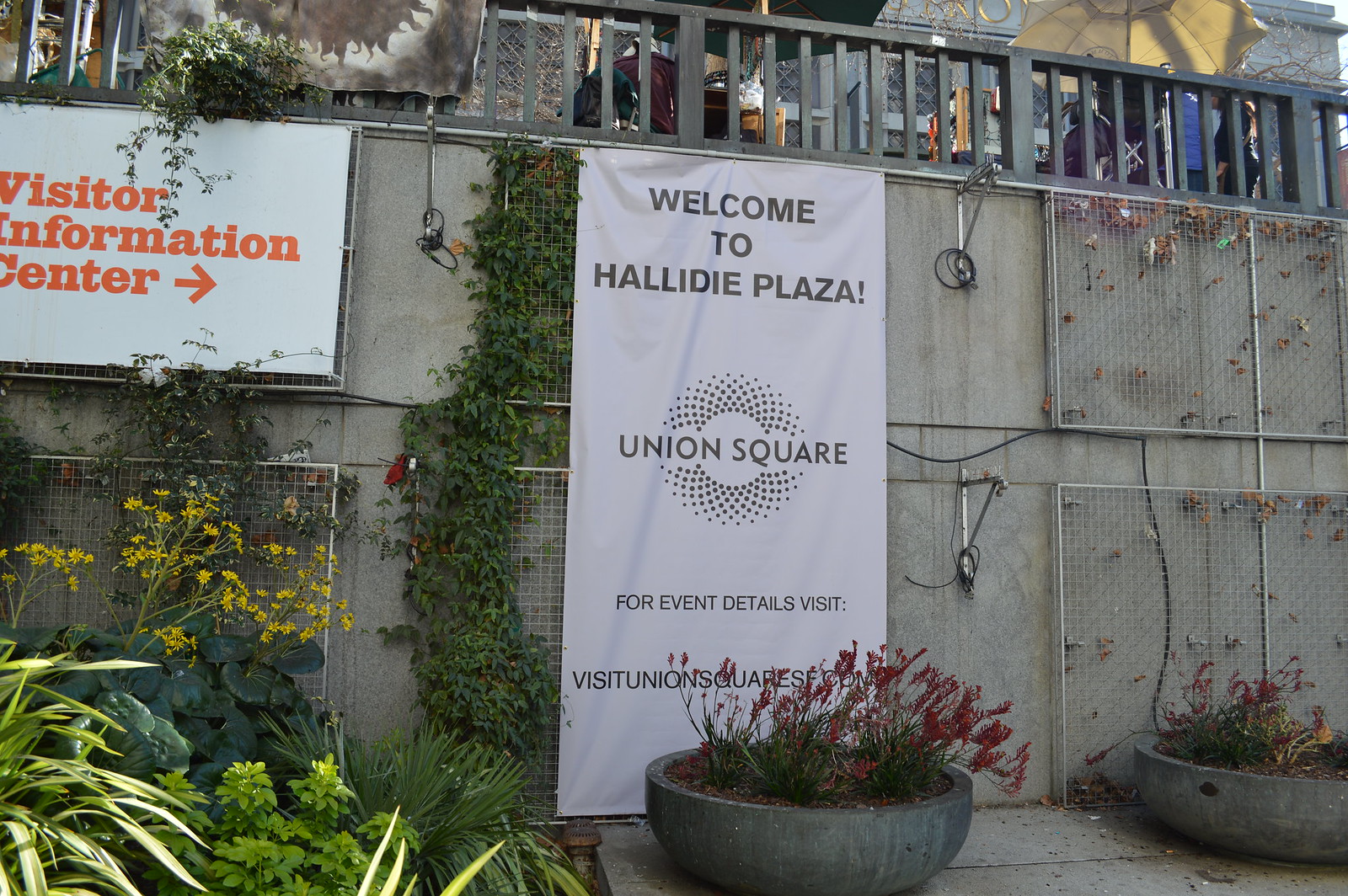The photograph captures the side of a two-story, gray stone building adorned with lush ivy and featuring a patio area on the second story. Prominently hanging from the wall, which also supports climbing plants through wire meshes, is a white vertical rectangular sign with black text that reads, "Welcome to Hallidie Plaza!" Below this main text is a spirographic logo with the label "Union Square," followed by a line stating, "For Event Details, Visit," leading to a website that is partially obscured by a large stone planter brimming with vibrant red bushes. To the left of this sign, a horizontal rectangular white sign with orange text declares, "Visitor Information Center," and points to the right. Below the signs and along the ground, numerous potted plants and flowerbeds add to the greenery. The upper section of the photograph reveals a decked area with chairs and umbrellas, bordered by a railing, hinting at an inviting spot where people are seated. The scene is well-lit, suggesting a bright, sunny day, though the side of the building remains comfortably in the shade.